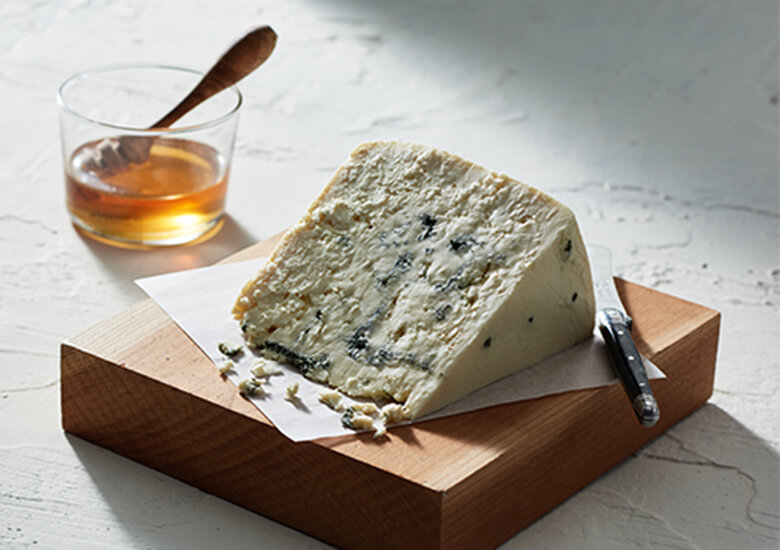The image features a detailed and artistic composition centered on a wedge of blue cheese. The cheese, speckled with blue and green mold, rests on a piece of white parchment paper. This parchment paper is placed on a light brown wooden cutting board. To the right of the cheese, a cheese knife with a black handle is partially visible, pointing away from the viewer. The knife is slightly covered by the cheese.

In the background on the upper left, there is a clear glass containing an amber liquid, likely honey. A wooden honey dipper protrudes from the glass. The tabletop surface beneath all of this is white and has a textured, spackled design. The illumination in the scene comes from the top left, casting shadows towards the bottom right, adding depth and contrast to the photograph. The overall setup is simple yet elegant, drawing attention to the detailed textures of the cheese, the honey, and the wooden cutting board.